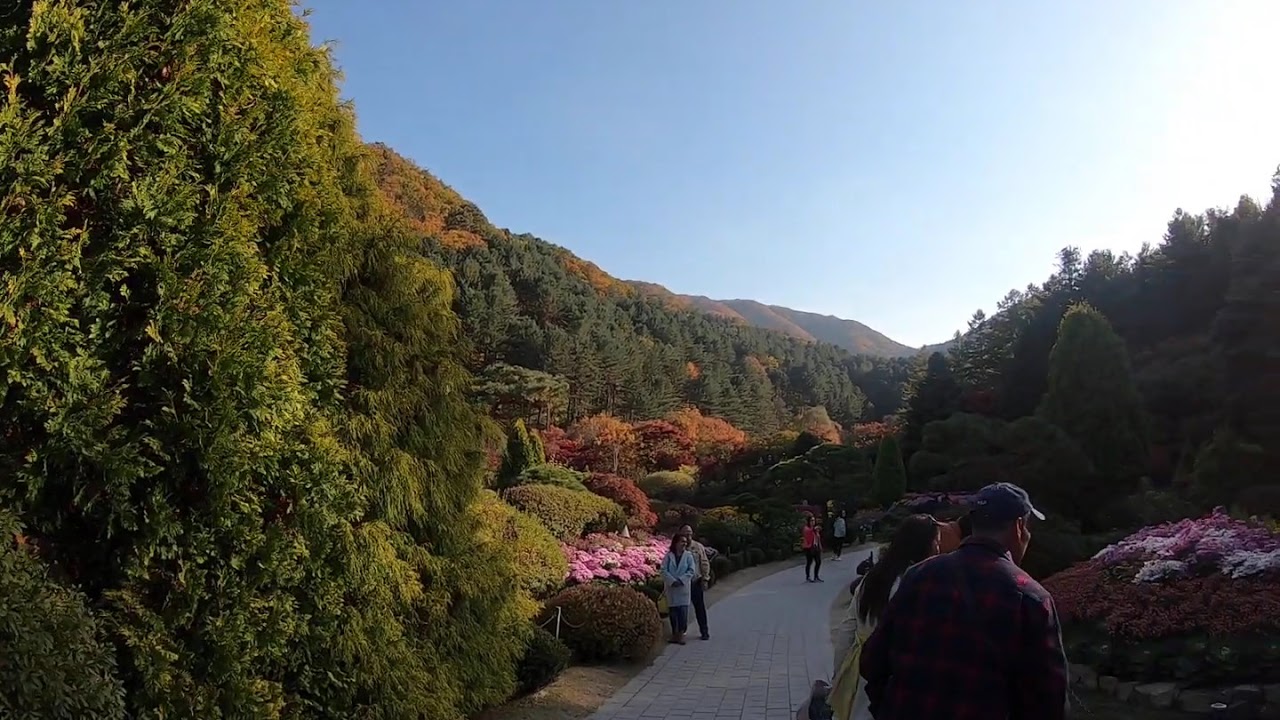The photograph captures a serene outdoor scene, likely a well-maintained garden set against a backdrop of lush greenery and rolling hills. A narrow stone path, wide enough for about four people abreast, runs through the center of the image. The path is flanked by meticulously tended flower beds, showcasing pink flowers on the left and a mix of pink and white flowers on the right. Several visitors, clad in fall attire including jackets and caps, stroll leisurely along the path, some stopping to admire the blooms. The surrounding area is densely forested with tall, lush trees and bushes forming a natural enclave around the garden. In the distance, the landscape transitions into rolling, forested hills, with the vibrant fall foliage of oranges, yellows, and reds contrasting against the muted hues of the distant trees. The sky overhead is clear, with the bright sunlight illuminating the scene from the right, casting a serene glow over the entire area. No buildings or structures are visible, allowing nature's beauty to take center stage in this idyllic setting.